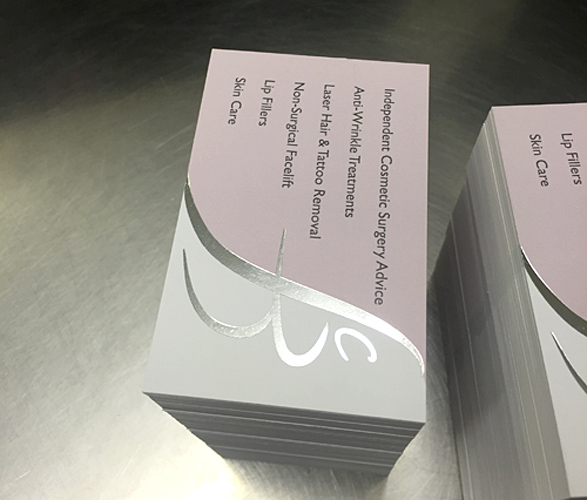The image appears to be an advertisement featuring two stacks of business cards set against an off-white surface. The prominent stack, located in the center of the image, displays a vertical orientation, with the cards angled to the left. They are visually divided, with a soft pink section on the left containing black text, and a silver detail on the right. The text on the cards includes multiple lines, reading: "Independent Cosmetic Surgery Advice," "Anti-Wrinkle Treatment," "Laser Hair and Tattoo Removal," "Non-Surgical Facelift," "Lip Fillers," and "Skin Care." The secondary stack of cards, partially visible on the right side of the image, repeats the same text and design elements. The cards feature a unique design with a silver motif, resembling a woman's silhouette or a stylized bee, in their silvery section. The overall feel of the cards is somewhat intricate and sophisticated, emphasizing cosmetic services without identifying a specific business or practitioner.